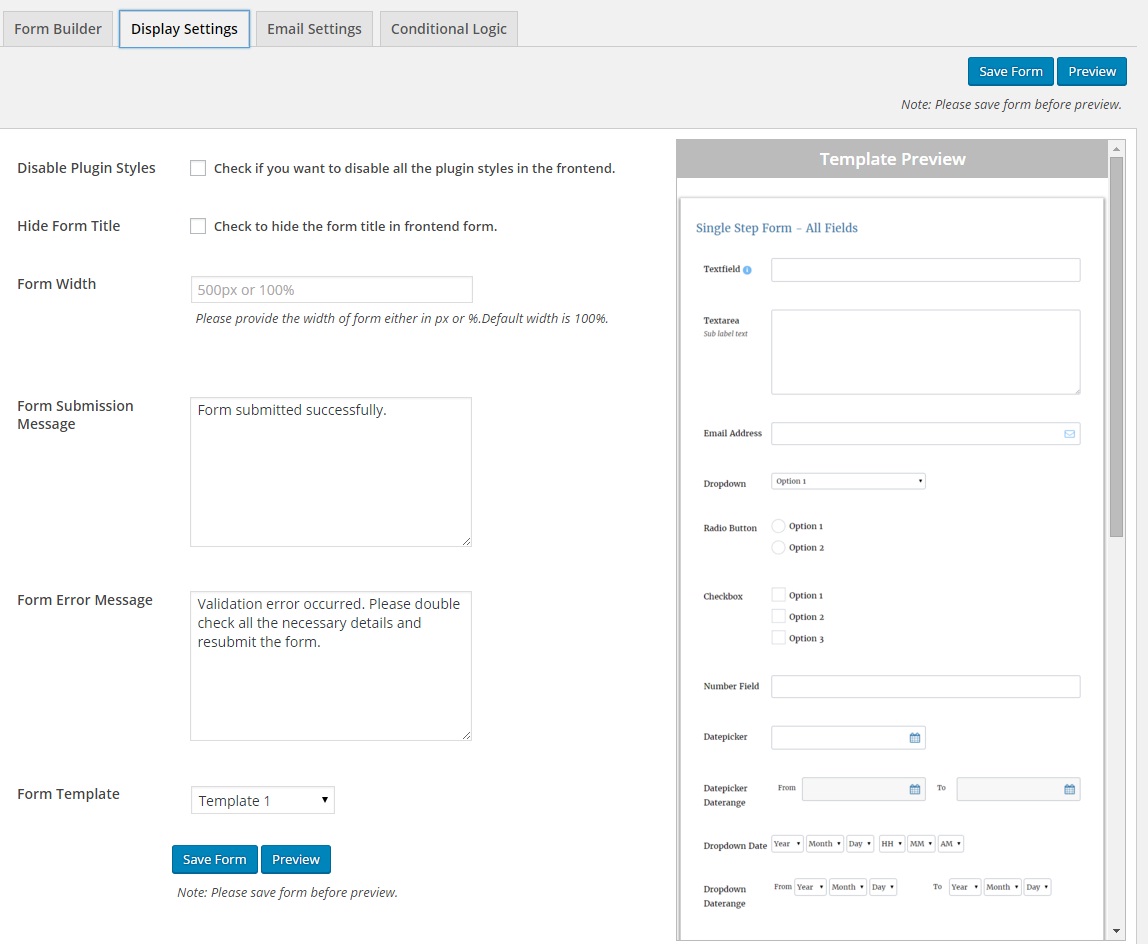**Image Description:**

The image displays the interface of a form builder application. The top section of the interface is predominantly gray, featuring a navigation bar with several tabs arranged from left to right labeled as "Form Builder", "Display Settings", "Email Settings", and "Conditional Logic". Just below this navigation bar is a gray horizontal line, and towards the far right, there are two blue buttons: "Save Form" and "Preview".

Beneath the gray line, there is a prompt in text stating, "Note: Please save form before preview," followed by another thin gray line. The background below these lines is white, containing various form-setting options.

On the left side, the options are listed vertically:

1. **Disable Plugin Styles**: A checkbox to disable all plugin styles on the front end.
2. **Hide Form Titles**: A checkbox to hide form titles on the front end.
3. **Form Width**: An input box for defining the width of the form, either in pixels or percentage, with the default set at 100%.
4. **Form Submission Message**: A text box for setting the message displayed upon form submission.
5. **Form Error Message**: A text box for configuring the message shown when there's an error with the form submission.
6. **Form Template**: A dropdown menu for selecting different form templates.

At the very bottom center of this white section, there is another blue button labeled “Save Form and Preview” with white lettering, accompanied by a reminder text underneath, reiterating to save the form before previewing.

To the right, positioned within a gray box, is a "Template Preview" section labeled "Single Form - All Fields". This section appears to list fourteen items (although the text is too small to read clearly), suggesting multiple fields to be filled out. At the very bottom of this sidebar, there is a dropdown box and possibly a pixel input option.

This detailed layout focuses on settings and customization options for creating and managing forms.